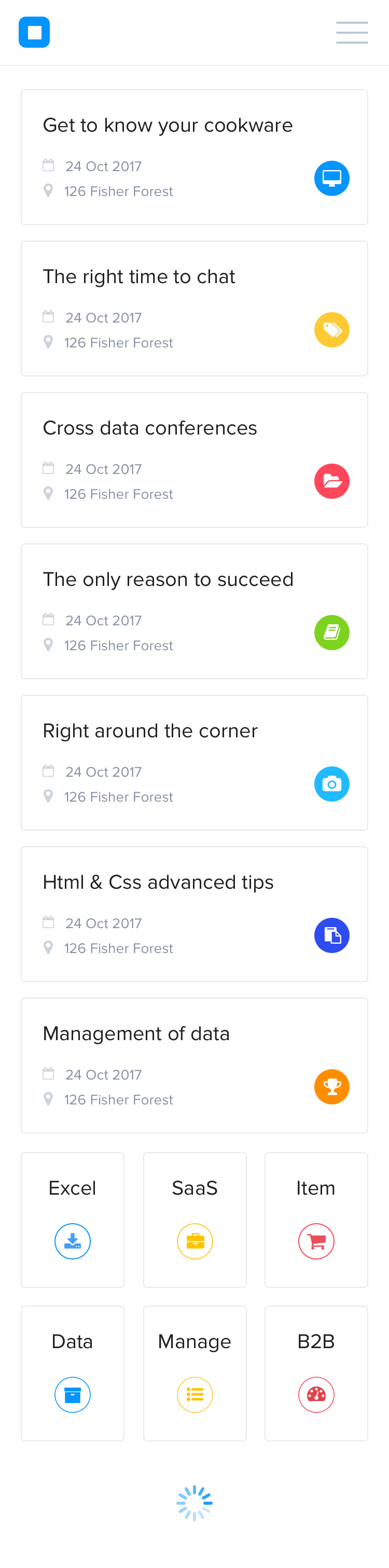**Screenshot Description:**

The screenshot captures a visually structured column of rectangular boxes aligned vertically, each representing distinct events or concepts. The layout begins at the top left-hand corner with a blue square enclosing a smaller white square. In the top right-hand corner, there are three thin gray vertical lines.

Each rectangular box conveys an event, all scheduled for the same date, October 24th, 2017, and location, 126 Fisher Forest. The events are listed as follows:

1. **Get to Know Your Cookware**
   - **Date:** October 24th, 2017
   - **Location:** 126 Fisher Forest
   - **Icon:** Monitor

2. **The Right Time to Chat**
   - **Date:** October 24th, 2017
   - **Location:** 126 Fisher Forest
   - **Icon:** Tag

3. **Cross-Stated Conferences**
   - **Date:** October 24th, 2017
   - **Location:** 126 Fisher Forest
   - **Icon:** Open Folder

4. **The Only Reason to Succeed**
   - **Date:** October 24th, 2017
   - **Location:** 126 Fisher Forest
   - **Icon:** Book

5. **Right Around the Corner**
   - **Date:** October 24th, 2017
   - **Location:** 126 Fisher Forest
   - **Icon:** Picture Symbol

6. **Hotmail and CSS Advanced Tips**
   - **Date:** October 24th, 2017
   - **Location:** 126 Fisher Forest
   - **Icon:** Chart with a Page

7. **Management of Data**
   - **Date:** October 24th, 2017
   - **Location:** 126 Fisher Forest
   - **Icon:** Trophy

Beneath these events, the screenshot includes six additional boxes arranged in a 3x3 grid. The content of the boxes from left to right and top to bottom are:

1. **Excel**
2. **SAAS**
3. **Item**
4. **Data**
5. **Manage**
6. **B2B**